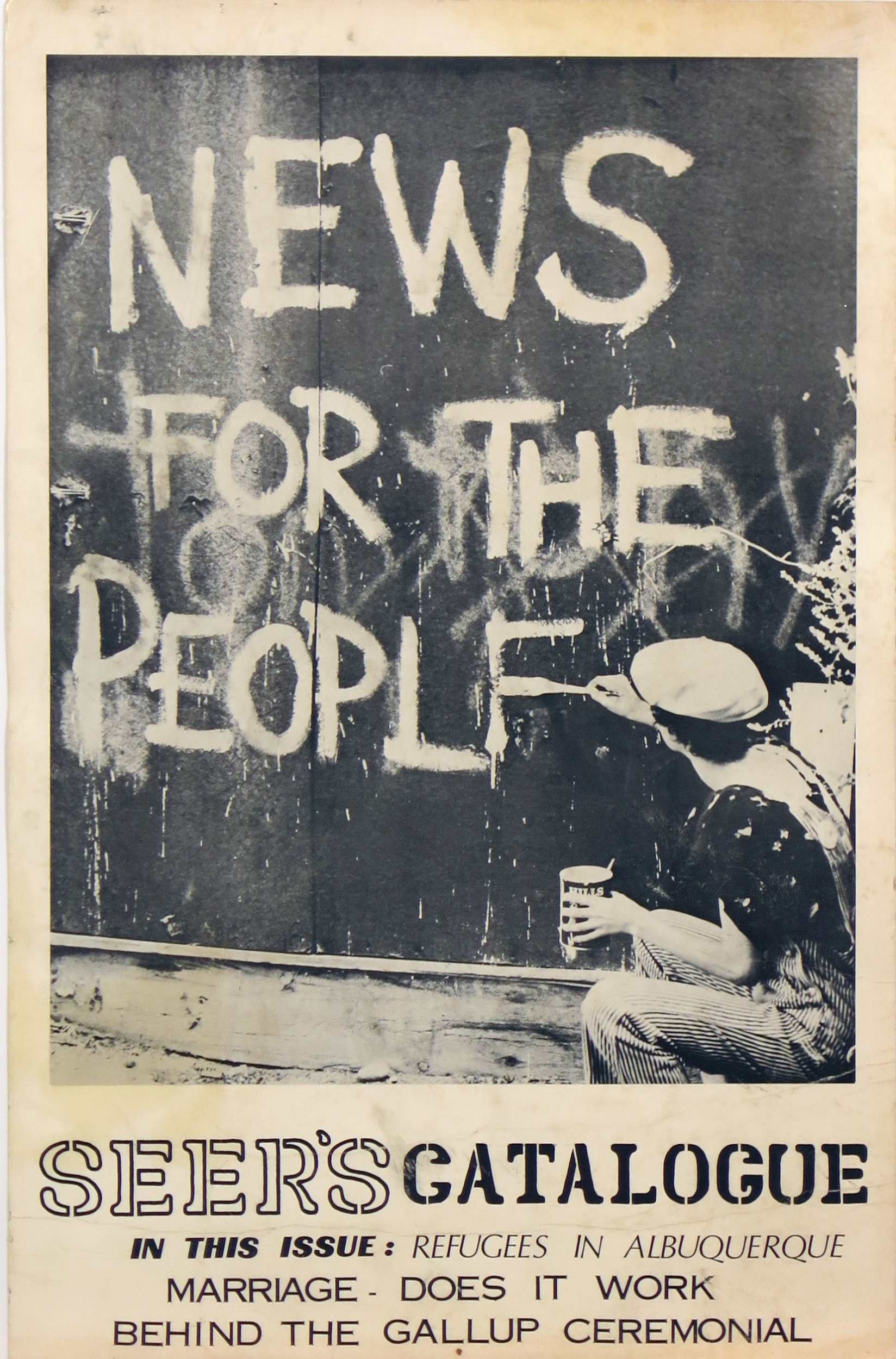The image depicts a weathered, tan-bordered poster that resembles an old, printed publication. Dominating the poster is a black-and-white photograph of a person in a scally cap and striped overalls, wearing a short-sleeved shirt. This individual, seen from a side view, is seated outdoors by a possibly sidewalk area, focusing intently on painting a black wall. The wall bears the partially completed white text, "News for the People," with only the letters "P-E-O-P-L" and part of the "E" visible. The painter is holding a brush in the right hand and a can in the left hand. Below the photograph, the poster reads "Sears Catalog." In smaller text, it lists the issue's contents: "refugees in Albuquerque," "marriage, does it work," and "behind the Gallop ceremony." The overall presentation gives it the appearance of being a vintage flyer or magazine cover.